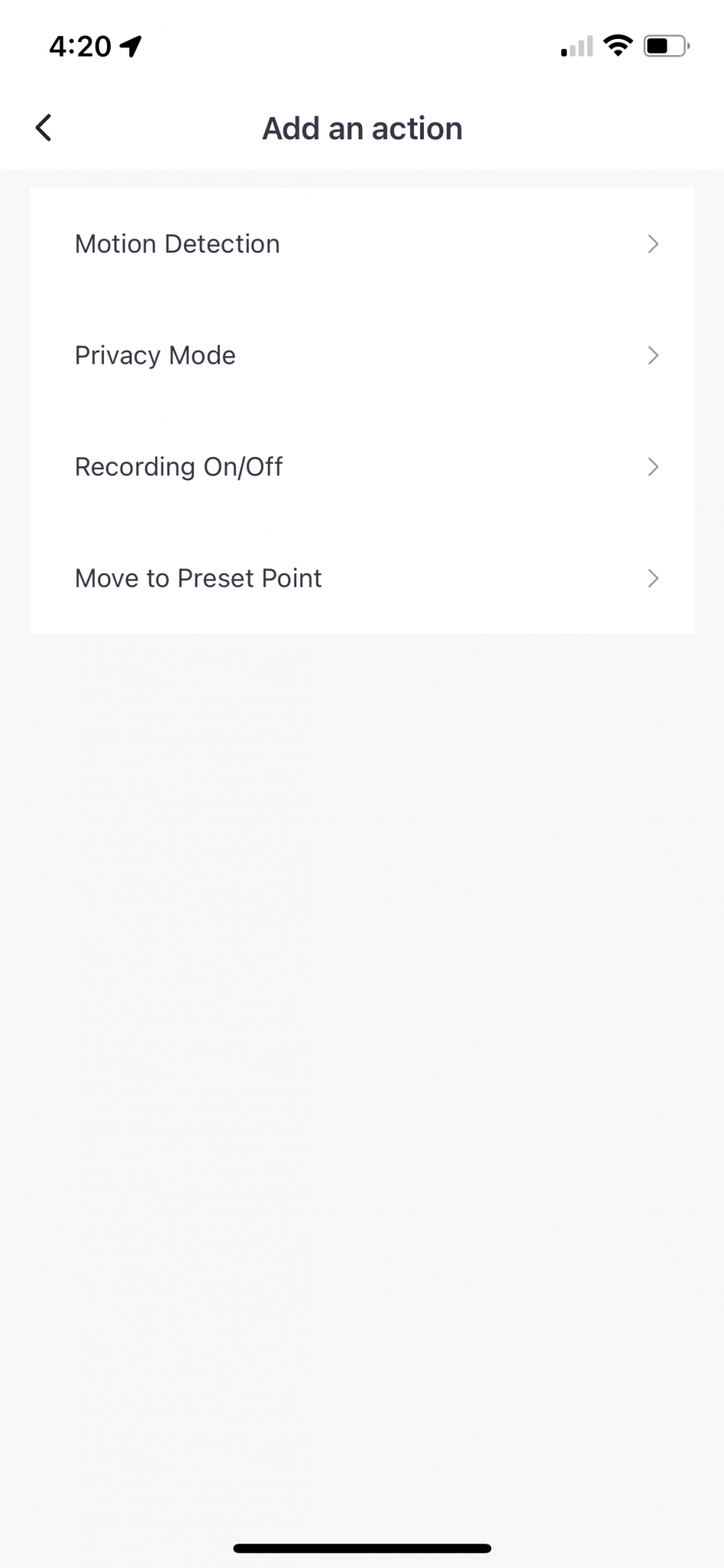This image is a screenshot of a smartphone with a white background. In the top left corner, the time reads "4:20," and there is a paper airplane icon for sending located just to the right of it. On the top right corner, there is a Wi-Fi icon showing only one out of four bars, next to the radar-like Wi-Fi signal icon. Adjacent to these icons is a battery symbol, indicating it is half full.

Dominating the center of the bottom section is the phrase "Add an action" displayed in bold black lettering. Above this, a left arrow is positioned on the left-hand side, which suggests a navigational option. Below the "Add an action" prompt, there is a list of four titles each accompanied by a right arrow on their far right side for additional actions:

1. Motion Detection
2. Privacy Mode
3. Recording On/Off
4. Move to Present Point

This list is set against a slightly lighter white background, bordered by an even lighter, almost white, edging that visually outlines the list within the overall white background of the screenshot.